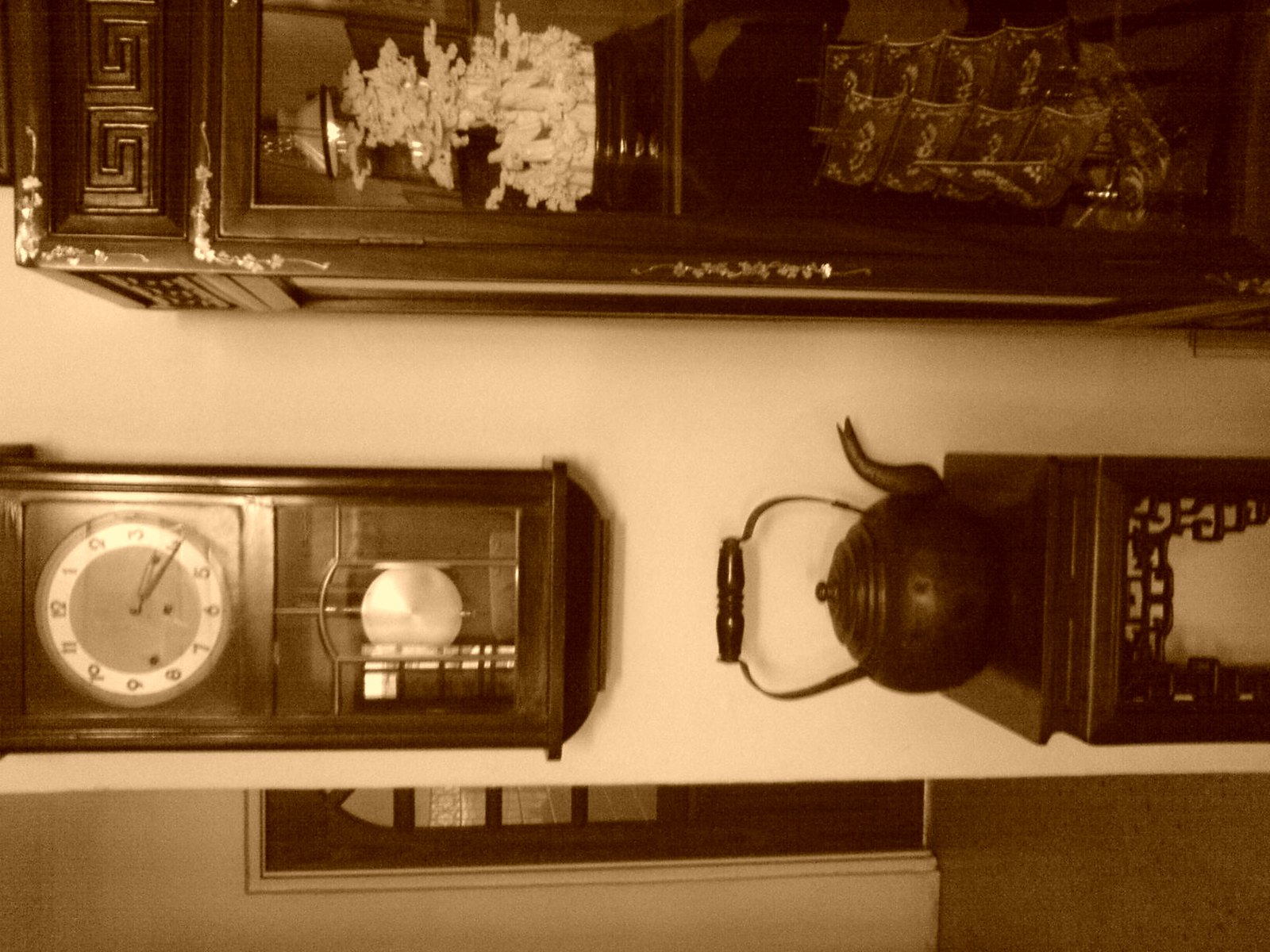This photograph, although oriented sideways to the left, features an antique, possibly Asian, curio cabinet filled with intricately carved figurines that appear to resemble trees. The top section of these figures is white, transitioning to a darker hue below. Centrally displayed in the scene is an old-fashioned pendulum clock with a wooden frame and a glass front, adding to the vintage aesthetic. Below the cabinet rests a small table, adorned with an old-fashioned iron kettle. To the left of the cabinet, the image captures a glimpse into an adjacent room, revealing a front door with glass panes that offer a view of a porch and a white wall beyond.